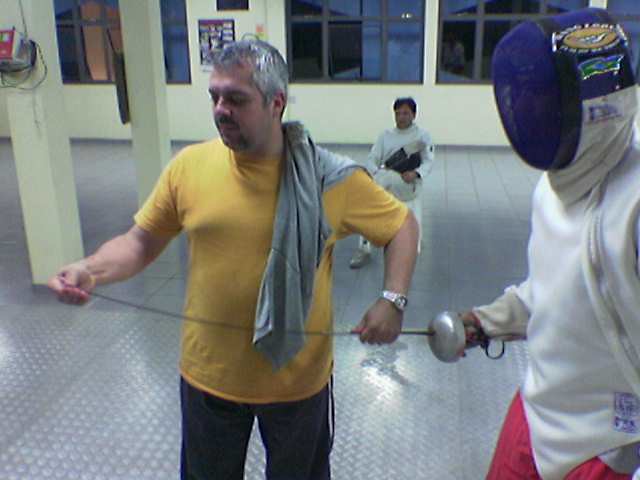In this detailed scene set within an indoor dojo that resembles a karate studio, a fencing lesson is taking place. The dojo, characterized by its gray, rubberized floor and pale green walls adorned with signage and windows overlooking a snowy exterior, is the backdrop for this intricate activity. 

At the center, a person, fully clad in traditional fencing attire that includes a white thick fabric suit and a blue mesh mask covering their face, stands poised yet not engaged in a fencing bout. The suit features a sensor embedded within to detect hits from the fencing sword. In the background, another individual similarly dressed in fencing gear, albeit without their mask, sits patiently in a chair. This person is wearing white attire paired with beige pants, sneakers, and is holding something in their hand.

Dominating the scene is a man who appears to be the instructor, distinguished by his silver hair. He is dressed in a yellow short-sleeve shirt and black Adidas-style sweatpants with a white stripe, with a long gray shirt draped over his shoulder and a gold watch on his wrist. This instructor is seen carefully inspecting or making adjustments to the tip of the foil held by the standing fencer, suggesting he may be providing some form of guidance or instruction.

The dojo's environment, with its striking white pillars and windows that let in natural light, creates an ideal setting for this engaging fencing lesson, capturing the meticulous nature of the sport and the attentive atmosphere of the training session.